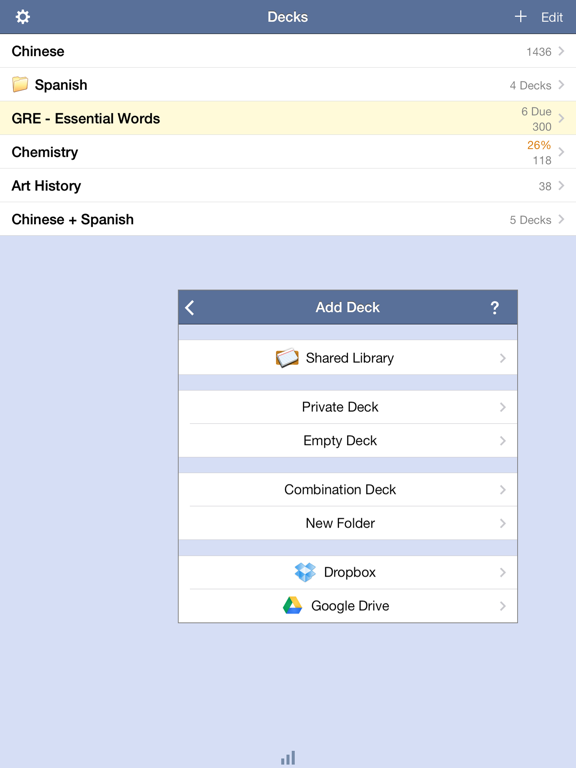The vertically oriented rectangular image showcases a user interface design, most likely for a digital flashcard or study application. The topmost section features a bluish-gray bar that spans the width of the page, containing a gear symbol on the far left, the word "Decks" centered, and a plus sign along with the word "Edit" aligned to the right.

Beneath this bar, the interface is divided into multiple sections, each separated by thin gray lines. The first section has a white background with black text. It starts with the word "Chinese" on the far left and concludes with "1436" on the far right, accompanied by a right-pointing arrow.

The next section below follows a similar format but begins with "Spanish" and includes a folder icon to the left of it. It mentions "four decks" and also has a right-pointing arrow.

The following section is highlighted in yellow, labeled "GRE - Essential Words," displaying "6 / 300" on the right along with a right-pointing arrow for further navigation.

Further down, the list includes "Chemistry" marked at "26%" progress and "118," followed by a right-pointing arrow. Another list item is "Art History," showing "38" and, you guessed it, a right-pointing arrow.

Subsequent entries mention combined categories such as "Chinese + Spanish" with "five decks."

Toward the bottom of the image, there is a lighter blue section which prominently features a pop-up window. This pop-up includes a dark blue banner at its top, containing the text "Add Deck" and a question mark icon on the far right. Within the pop-up, additional words and input options are present, further enhancing the user interactivity of the interface.